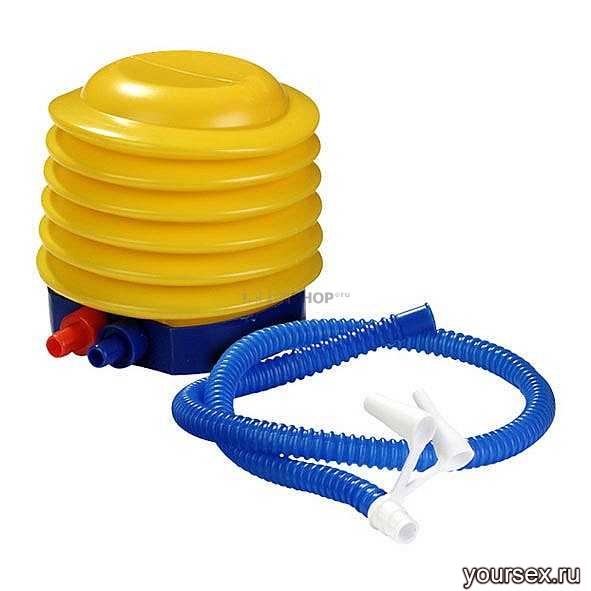The image features a disassembled children's toy pump, meticulously laid out against a solid white background. The main component on the left is a vertical, yellow flexible pump structure with a red nozzle and a dark blue base, which also houses a blue nozzle. These nozzles are potentially for intake and output of air. Adjacent to this, on the right, is a coiled blue tube with ridges and a white cap at the end, along with additional blue caps. The objects are well-centered and presented diagonally, spanning almost the entire frame to reveal all parts clearly from a side angle. The photograph has a watermark that reads "hop" and a URL at the bottom right corner, "yoursex.ru", displayed in white letters with a black outline. The colors predominantly include blue, yellow, white, red, and a hint of gray, with the items suggesting functionality related to air transfer, likely in a retail product setting.